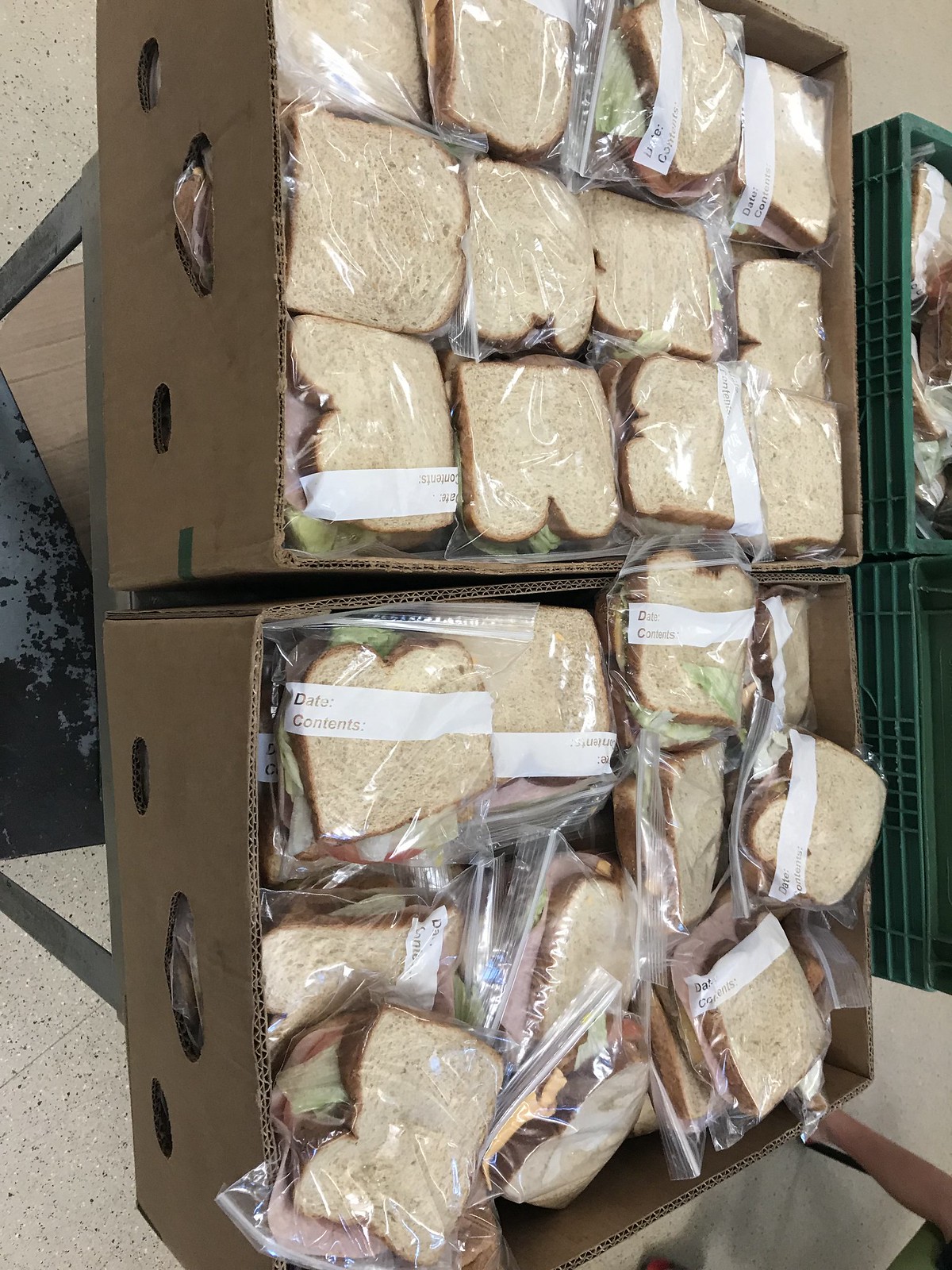The image presents a cluttered scene captured at a sideways angle, focusing on two large, brown corrugated cardboard boxes resting on a tipped-over metal platform atop a marble countertop. Each box is filled with sandwiches wrapped in plastic Ziploc bags. The sandwiches, neatly stacked in one box and scattered messily in another, are made of either whole wheat or white bread, containing cheese and lettuce, with some possibly including ham. The plastic bags have a white strip at the top, presumably for labeling. The boxes, which feature oval-shaped holes for handles, are positioned in the center of the photograph. Behind them, to the right, a stack of green plastic crates is visible, perched against a wall. Chrome legs of the table supporting this setup can also be seen, along with part of a person's leg seated on a green chair in the background.